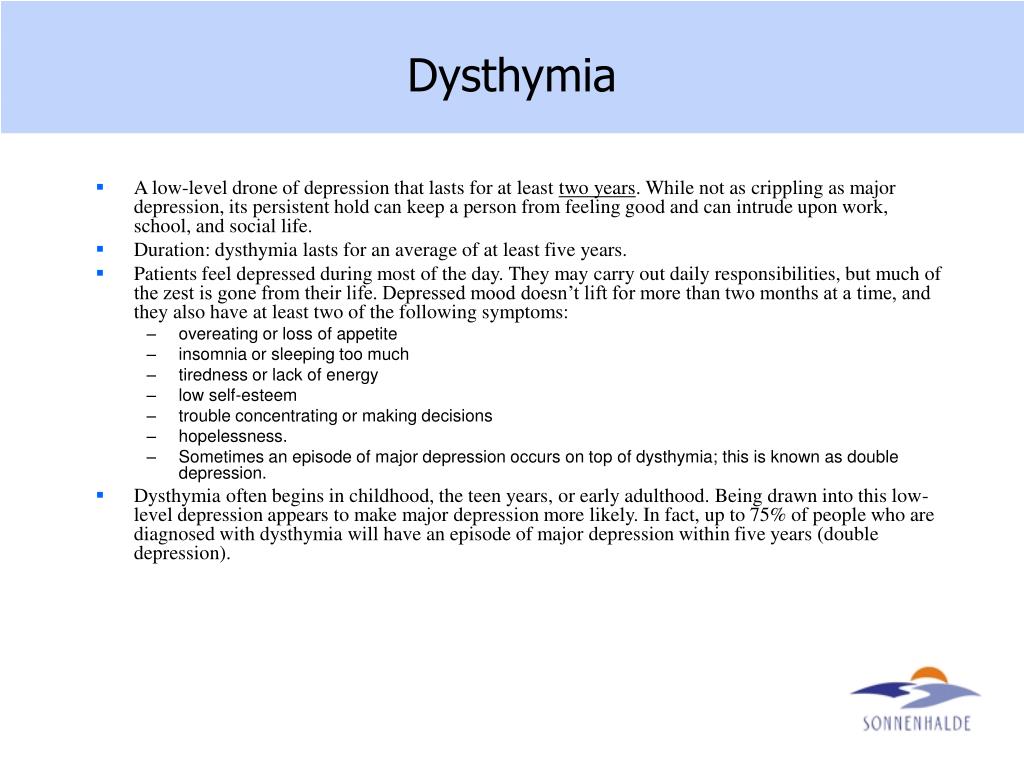**PowerPoint Slide on Dysthymia**

**Dysthymia (D-Y-S-T-H-Y-M-I-A)**

**Overview:**

- Dysthymia, also known as Persistent Depressive Disorder, is characterized by a low-level, chronic form of depression that lasts for at least two years (with the duration of "two years" being specifically underlined).
- Although not as debilitating as major depression, its persistent nature can significantly affect one's quality of life, interfering with work, school, and social interactions.

**Duration and Symptoms:**

- **Average Duration:** Dysthymia typically persists for a minimum of five years, with patients feeling depressed most of the day.
- **Daily Function:** While individuals may still perform daily responsibilities, the zest and enthusiasm for life are markedly diminished.
- **Symptom-Free Periods:** The depressed mood does not fully lift for more than two months at a time.
- **Additional Symptoms:** At least two of the following symptoms are present:
  - Overeating or loss of appetite
  - Insomnia or hypersomnia (sleeping too much)
  - Fatigue or lack of energy
  - Low self-esteem
  - Difficulty concentrating or making decisions
  - Feelings of hopelessness

**Double Depression:**

- **Development:** An episode of major depression can occur in conjunction with dysthymia, a condition referred to as "double depression."
- **Onset:** Dysthymia often begins during childhood, adolescence, or early adulthood.
- **Progression:** Those with dysthymia are more likely to develop major depression, with up to 75% of individuals experiencing an episode of major depression within five years of their dysthymia diagnosis. 

This slide provides a comprehensive overview of the persistent depressive disorder known as dysthymia, highlighting its symptoms, duration, and potential progression to more severe forms of depression.